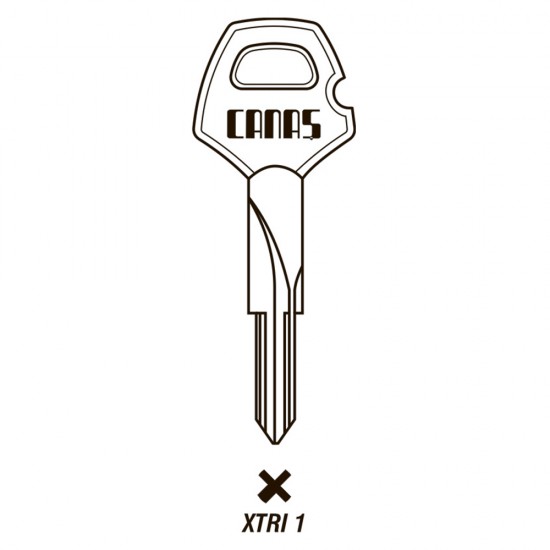This is a simple, two-color black and white illustration of a key. The key is rendered in white with a black outline, standing vertically in the image. The handle, located at the top, features the word "CANAS" (C-A-N-A-S), which appears in capital, futuristic lettering. The handle has a pentagon shape with an oval-shaped hole for a key ring and a small semicircular notch on the right-hand side. The shaft of the key extends downward, devoid of teeth, and has two switches leading to the tip, which narrows towards the bottom. Below the tip of the key is a prominent thick black X. Further underneath, there's text that reads "X T R I 1," with the characters aligned diagonally to the right. The lower half of the key’s shaft is adorned with vertical lines, adding to its unique design.